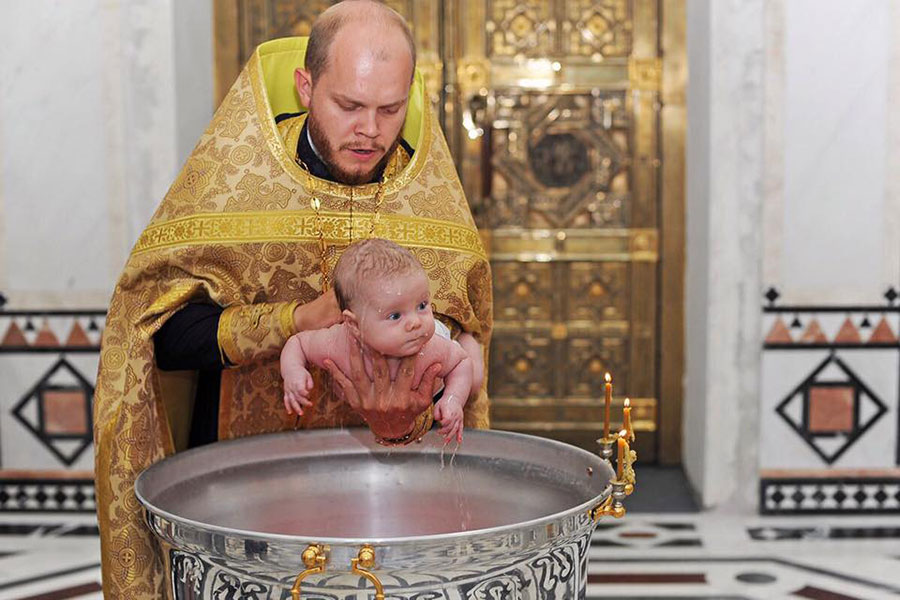In the image, a baby is being baptized by a priest, possibly from a Russian or Greek Orthodox Church given the ornate gold cloth he is wearing, which differs from typical Catholic vestments. The priest holds the baby's chest with his open hand, tilting the baby face down over a bowl of holy water for the baptism. The baby, appearing wet and slightly distressed from the immersion, looks to the right. The priest, adorned in a highly elaborate gold robe with intricate designs, seems slightly nervous as he conducts the ritual. Behind them, there are lavishly decorated doors, likely made of or plated with gold, accompanied by detailed marble or tiled floors and walls that feature complex patterns, including black lines and brown hues. Adding to the solemn atmosphere, lit candles are seen beside the basin used for the baptism. The overall setting exudes a rich, traditional church ambiance with its vivid, elaborate decor.